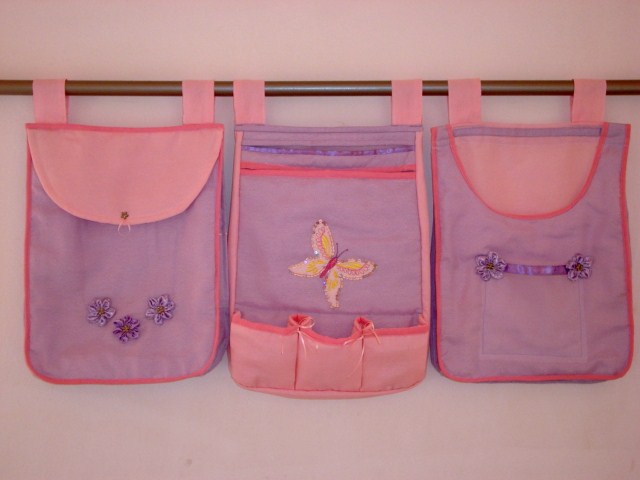The image showcases three small, likely handmade or custom-sewn, pink and purple pouches hanging vertically from a wooden rod against a pale pink or dark pink wall. The rod is positioned horizontally near the top of the image, resembling a curtain rod. Each pouch has a distinct design but shares a child-like aesthetic with purple bodies and pink flaps or trims. The leftmost pouch features three purple flowers on its purple body and a pink flap. The center pouch, characterized by a yellow butterfly with a red body, includes multiple small pink pockets at the bottom and a pink stripe at the top. The rightmost pouch mirrors the first with a purple body, a pink flap, and additional flowers on the pocket. Each pouch is suspended by short pink straps, laying flat over the rod, maintaining a consistent rectangular shape with dimensions approximately in a three-by-two ratio, longer in height than in width.